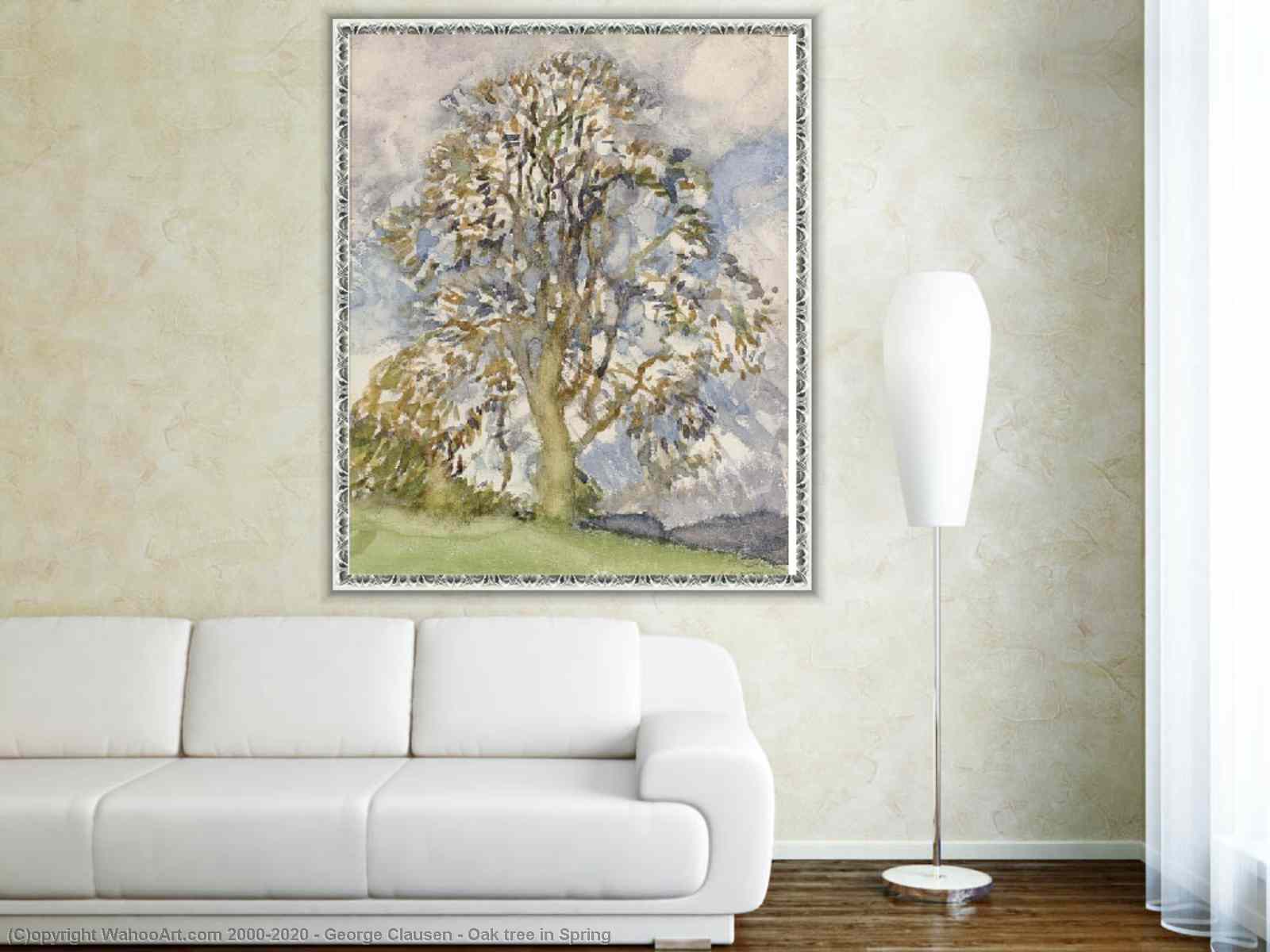This photograph captures a quaint living space that harkens back to the 1990s, with a touch of modernity. Dominating the room is a plain white sofa, potentially crafted from smooth leather or faux leather material, notable for its low-sized arms and backrest. Despite one description suggesting multiple cushions, the prevailing view is that the sofa stands bare, emphasizing its sleek, minimalist design. The floor beneath is a richly glossed brown wooden surface, contributing to the room's vintage charm. Positioned strategically beside the sofa is a tall, freestanding lamp featuring a large white lampshade and a vertical pole, casting a warm glow across the space. The backdrop is a light tan wallpaper, against which hangs a prominent watercolour painting of a large oak tree in spring. The artwork, attributed to George Clausen and spanning from 2000-2020 as indicated by the digital watermark 'WahooArt.com,' showcases a serene landscape with the oak tree standing majestically against a vividly blue, cloud-swirled sky, accompanied by green hills and distant bushes. This careful composition suggests the photograph's purpose is to highlight the timeless beauty of the Clausen painting within a thoughtfully curated domestic setting.